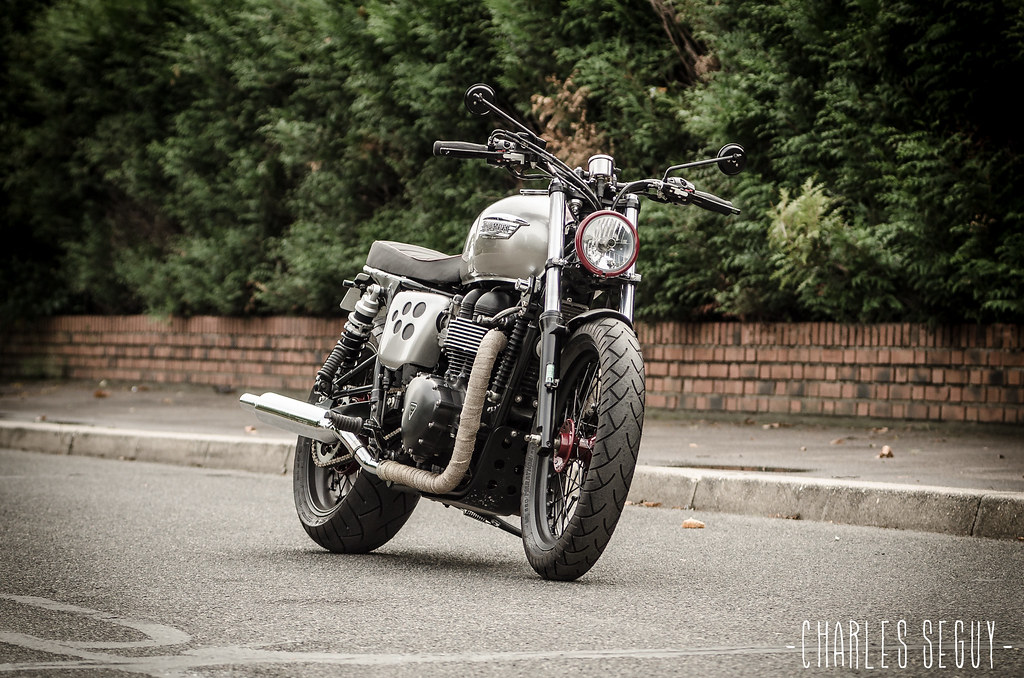The image depicts a dark black motorcycle parked in the middle of a light brown paved street. The motorcycle is leaning to its left with the kickstand down. It features a silver gas tank, dark black handlebars, and a black seat. The front tire is visible, bolstered by the headlight with a red rim and mirrors extending from it. In addition, a tube-like feature runs from behind the front tire to the back tire, which is also visible. 

In the background, a short orange brick wall, approximately two feet high, stretches horizontally across the midpoint of the image. This wall is accentuated by a sidewalk running from left to right, with a white stone curb marking its edge. Behind the brick wall lies a dense, impenetrable mass of green bushes and trees, creating a backdrop of thick foliage. The photograph is rectangular and horizontal in orientation. In the bottom right-hand corner, the text "Charles Seaguy" is visible.